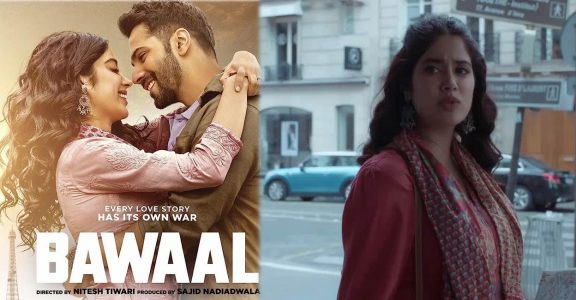The image features a composite of two visuals. On the left side, it showcases the front cover of the Indian movie "Bawal." The cover portrays a light-skinned Indian couple in an intimate embrace, gazing deeply into each other's eyes. The woman, positioned on the left, has long, curly black hair and is adorned in a purplish top, with noticeable earrings adding to her look. The man, standing on the right, has black hair, a neatly trimmed beard, and is dressed in an olive green shirt, with a hint of a blue dress shirt collar visible underneath. Below this tender scene, the text reads: "Every love story has its own war." The film title "Bawal" appears prominently, followed by credits stating it's directed by Nitesh Tiwari and produced by Sajid Nadiadwala. On the right side of the image, there’s a still from the movie showing a woman, likely the same as the one on the cover, standing on a city street in front of a building. She is captured mid-speech, wearing a red jacket with a scarf, her curly hair cascading around her face, with brown pedestrian signs visible in the background to her upper right. She's facing forward, her gaze directed away, adding a dynamic element to the composition.